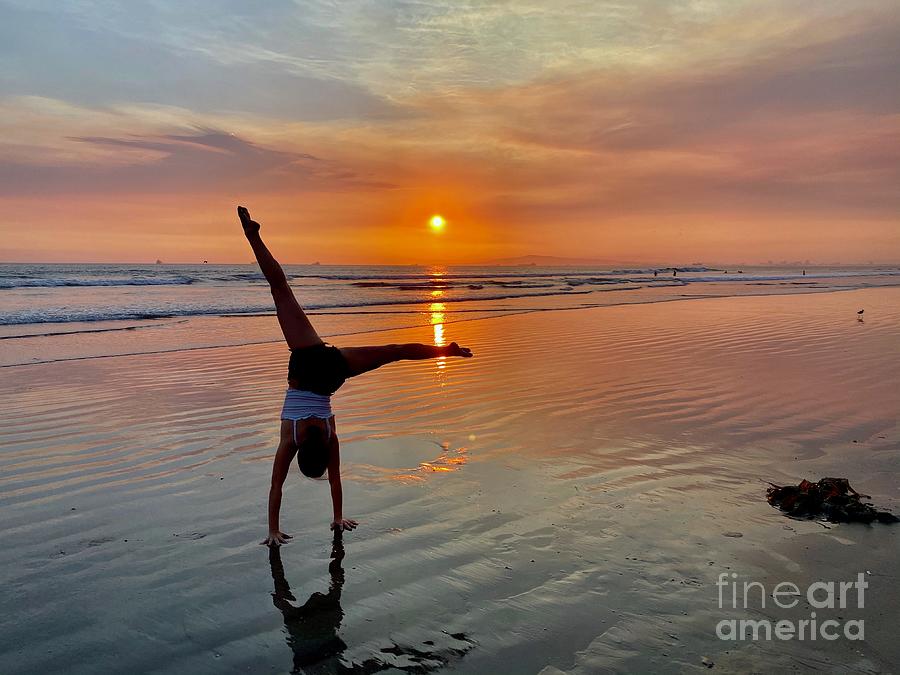This photograph captures a serene beach scene at sunset, with the sky transitioning from purple to pink and dotted with light clouds. The sun, positioned centrally, emanates an orange glow that reflects off the calm ocean waves, leading up to ships anchored on the horizon. The smooth, tan-colored beach is still wet from the receding tide, adding a glistening effect under the sun's rays. In the foreground, a woman with brown hair performs a handstand, her legs scissored towards the sun. She is barefoot, dressed in a white halter top and black, or possibly dark blue, shorts. There's some seaweed in the lower left corner and a few rocks and a bird to the right, with a few distant figures standing at the water's edge. The lower right corner of the photo features a light watermark reading "Fine Art America."